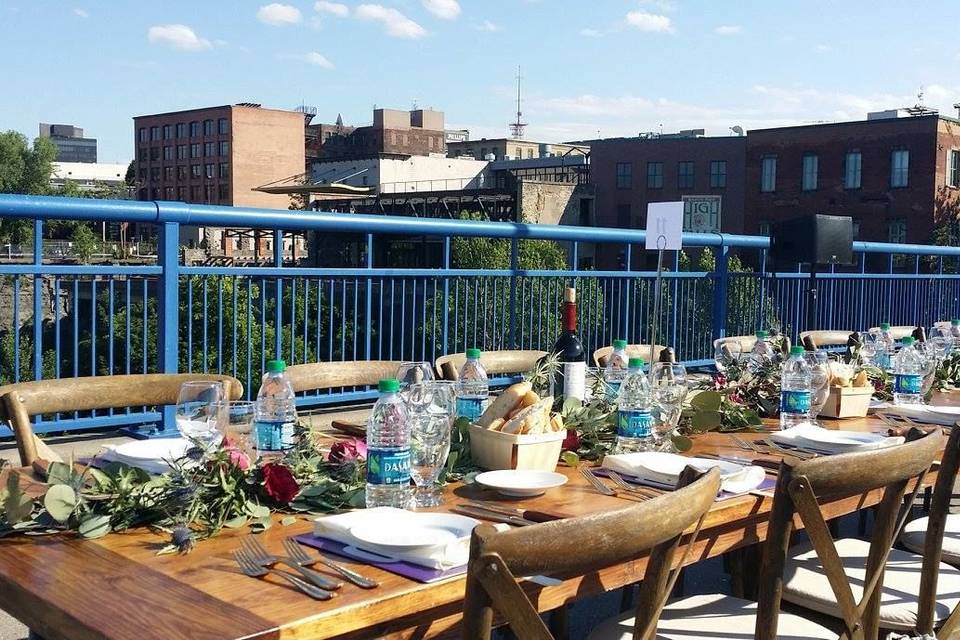The image captures a picturesque rooftop dining area, set several stories high amidst an urban landscape of brownstone buildings ranging from 6 to 10 stories tall. The outdoor setting is under a brilliant midday sky dotted with a few scattered clouds. A wooden table, running diagonally from the front left to the back right of the viewer, is elegantly arranged with empty place settings that include cloth napkins, plates, an array of silverware featuring three forks and two knives per setting, and a clear glass at each spot. Complementing the formality, a bottle of water and a bread basket are positioned at each place, alongside a casually arranged floral display of roses scattered between the items. The table is framed by a sturdy blue rail, beyond which trees and further cityscape details can be discerned. Wooden chairs encircle the table, each adorned with thin tan cushions tied to their backs, adding to the inviting atmosphere of this rooftop dining experience.